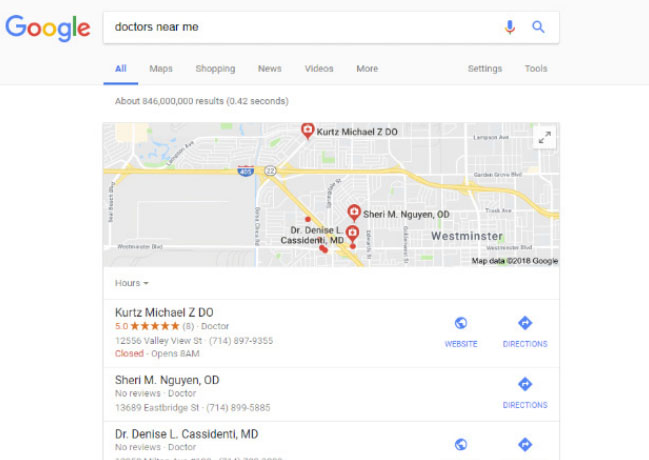The image is a screen capture of a Google search result page. At the top of the image, the recognizable Google logo is prominently displayed in its signature colors of blue, red, gold, and green. Directly beneath the logo is a search box containing the phrase "Doctors Near Me." Additionally, there is a red, gold, and blue microphone icon and a blue magnifying glass icon adjacent to the search box.

Below the search box, there are submenus with various options for refining the search. The submenu labeled "All" is highlighted in blue, while the others—Maps, Shopping, News, Videos, More, Settings, and Tools—are grayed out.

Further down, the number of search results and the time it took to generate the search are displayed. Beneath this information, a Google Maps view from what appears to be 2018 shows several businesses marked with red location pins, each featuring a small medical symbol. Notably marked locations include Kurtz Michael ZDO, Sherry M. Nygan OD, and Dr. Denise L. Castetti MD.

The search results are listed as follows:

1. **Kurtz Michael ZDO**
   - Rating: 5 stars from 8 reviews
   - Address: 12556 Valley View Street
   - Phone Number: 714-897-9355
   - Status: Closed, opens at 8 AM
   - Options: Website and Directions links, both in blue

2. **Sherry M. Nygan OD**
   - No reviews
   - Address: 13689 Eastbridge Street
   - Phone Number: 714-899-5885
   - Options: Directions link in blue (No website listed)

3. **Dr. Denise L. Castetti MD**
   - No reviews
   - (Address and phone number not fully visible as the bottom of the image is cut off)
   - Options: Globe icon presumably for the website and a Directions arrow icon

The bottom part of the image cuts off part of Dr. Denise L. Castetti's details, leaving some information incomplete.